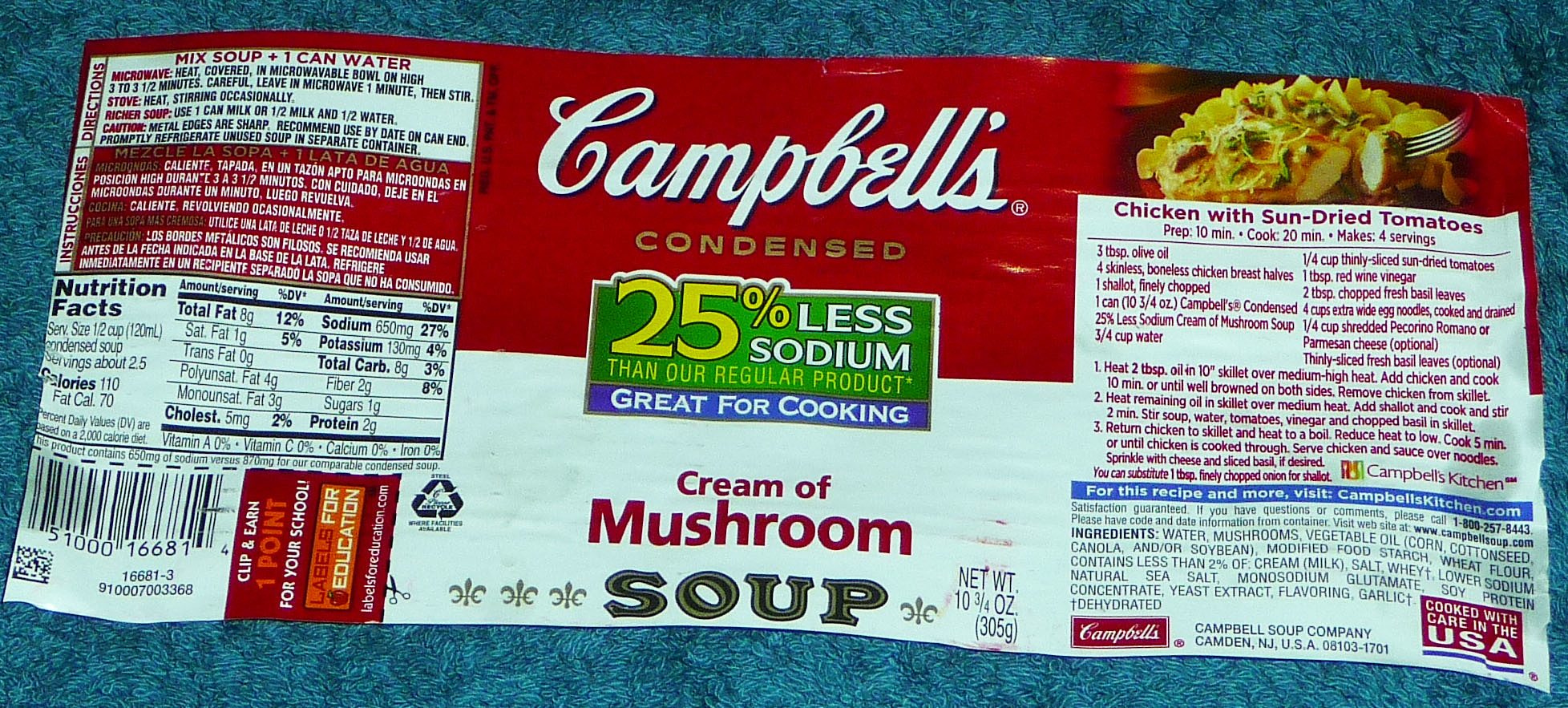This is a detailed photograph of a Campbell's soup label that has been removed from a can and laid out flat on a blue tabletop. The label, primarily red in color, features the iconic Campbell’s logo in white cursive lettering with a red background. This particular label is for condensed cream of mushroom soup and prominently displays a message in the center stating “25% less sodium than our regular product” along with “Great for cooking” in blue.

On the left side of the label, you can find the nutritional facts and instructions for preparing the soup, which include mixing the soup with one can of water and directions for both microwave and stovetop cooking, written in both English and Spanish. Additionally, this section hosts the UPC barcode needed for scanning and lists the ingredients with a blue line separating them for clarity. 

The right side of the label features a recipe for chicken with sun-dried tomatoes, accompanied by a picture of the dish. The label also notes that the product is made in New Jersey, USA.